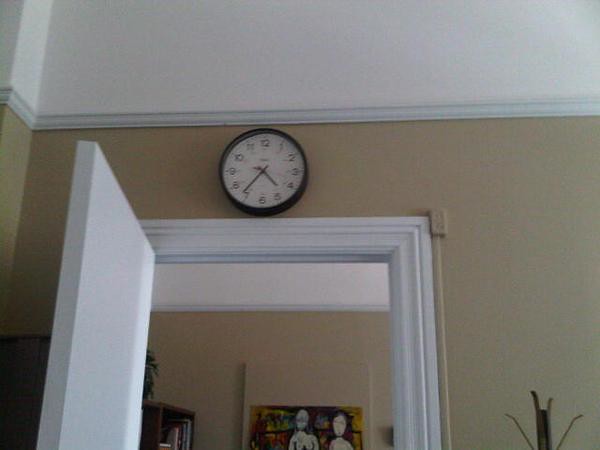This image prominently features a clock mounted on a wall within a high-ceilinged house. The wall is divided into two distinct color sections: the upper portion is a crisp white, while the middle to lower segment is a light tan color. The clock is centered on the dark tan part of the wall, positioned just above the white framing of a doorway. The clock itself is a modest size, approximately four inches in diameter, with a black circular border. The clock face displays numbers from 1 to 12, though only the numbers from 1 to 11 are visible in the upper left corner of the image. The shorter hour hand is pointing just above the 5, while the longer minute hand is slightly past the 7. Below the clock, there is a white doorway; to the left of the doorway is another white door that leads into an adjacent room. Visible beyond the doorway, there is another section of the wall adorned with a framed picture.